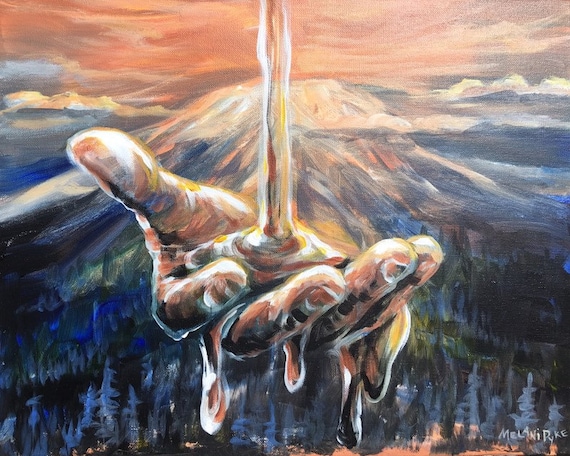The image is an elaborate, multicolored illustration that captures a surreal and vivid scene. Dominating the foreground is a large, detailed right hand, palm up, depicted in swirling shades of browns, whites, and dark grays. The light brown fingernails are clearly visible, adding to the hand's intricate realism. Liquid, possibly syrup or water, pours into the hand from the top of the picture, pooling in the palm before dripping through the slightly spread fingers onto the landscape below.

This hand emerges from a striking mountain that forms the background, a snow-covered peak reflecting colors from a vibrant sky. The mountain, reminiscent of Mount St. Helens viewed from its non-crater side, showcases hues ranging from gold to reddish-yellow at the top, blending into blues and greens. At its base, visibly lined with dark evergreen trees and patches of forest foliage, lies a valley with ground tones of gray and reddish ochre.

The sky itself is a mesmerizing tableau of sunset colors predominantly featuring oranges, but also incorporating pinks, blues, greens, and yellows, with additional mountains and clouds faintly visible in the distance. The entire scene exudes a dreamlike quality, further accentuated by a subtle blue image on the ground near the base of the trees, suggesting a body of water or part of the terrain.

In the lower right corner of the painting, the artist's name, Melanie Reich or Malini Rikki, is elegantly inscribed, solidifying the artwork's authenticity and unique style.